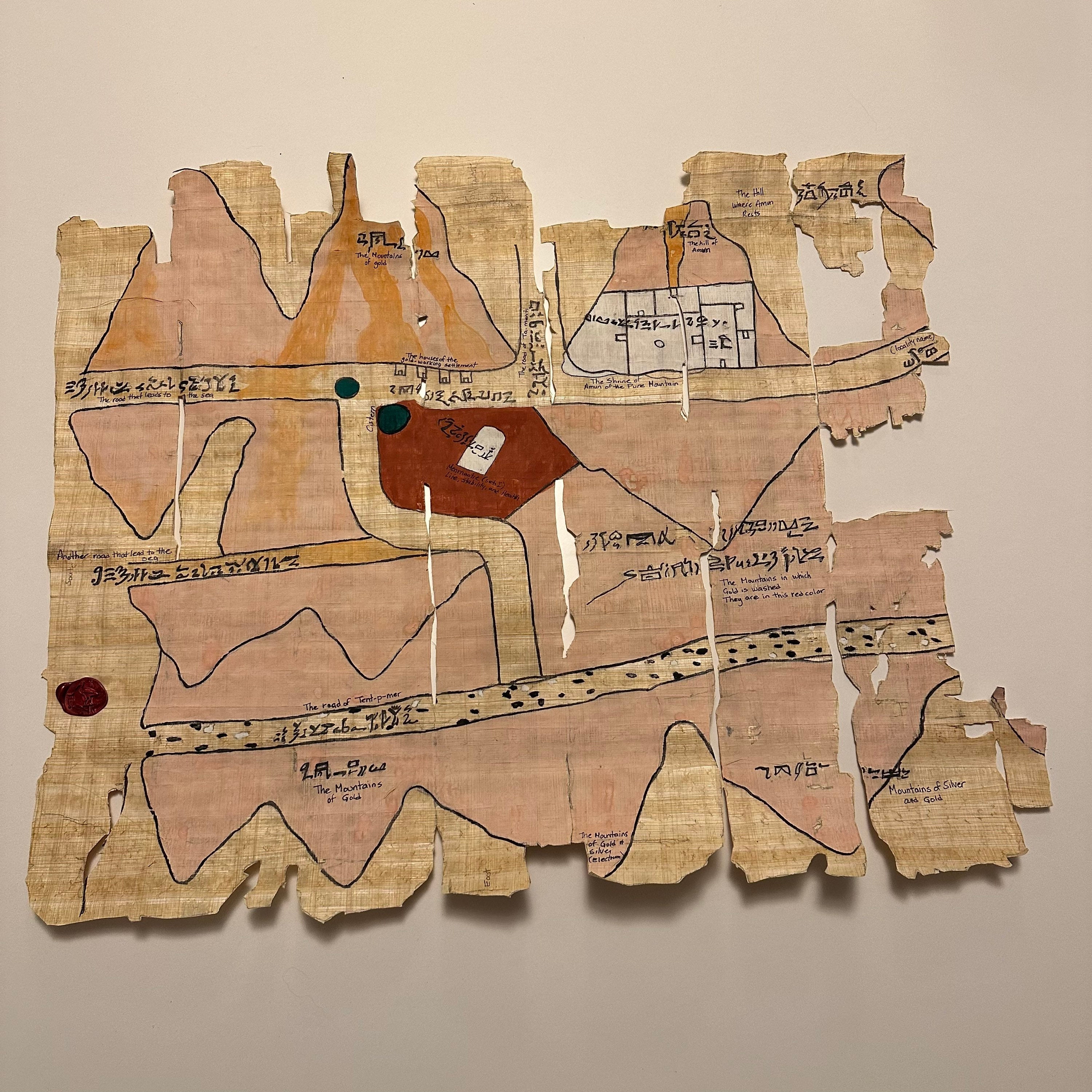The image depicts a tattered and ancient map, delicately drawn on what appears to be a cloth-like or papyrus material. The map exhibits jagged, worn-out edges, suggesting significant age or deliberate distressing. The background of the map is a tan hue, possibly resembling thick paper or aged wood, with a weathered consistency. The surface is marked by intricate black lines, creating unique patterns that divide the map into various sections. Among these divisions, you can discern shapes resembling mountains, painted in light and dark brown shades. Notably, a prominent dark brown area occupies the center, and a white rectangle is visible near the top section. The map also features unreadable symbolic writings, with legible inscriptions at the bottom stating "Mountains of Gold" and "Mountains of Silver and Gold." Additionally, it illustrates possible pathways, resembling roads, weaving through the depicted landscape.